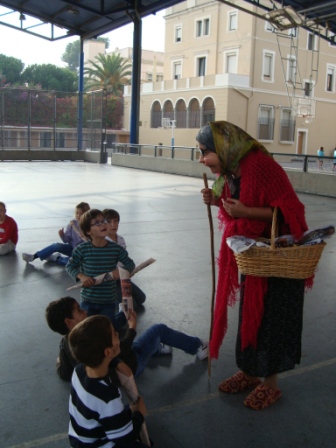The image depicts a scene, likely set in the daytime, featuring a woman in a long red dress and a shawl walking towards a group of young children. The woman holds a long walking stick in her right hand and carries a basket under her left arm. The basket appears to be filled with something indistinguishable. The children, all around four to five years old and primarily boys, seem very focused on the woman. The scene is set near a two to three-story building, which is partially visible in the background along with some bars and a fence, possibly indicating a playground or school area. The ground appears to be cemented and gray.